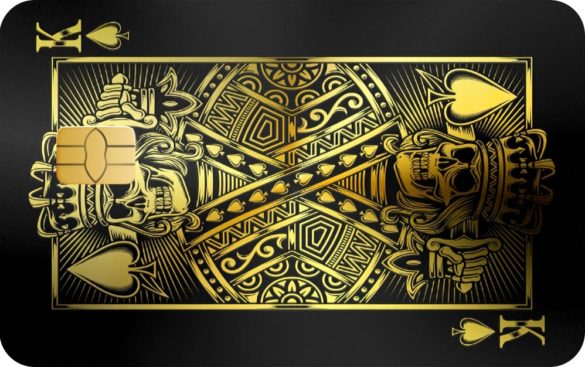The image is a photograph of a credit card designed to resemble a king of spades playing card. The card is horizontally oriented, featuring rounded corners and a solid black background. The intricate gold graphics depict two skeletal kings wearing crowns and holding swords behind their heads. Positioned on the left and right, each king has a skeletal face and dons armor adorned with various geometric shapes, including spades. The distinguishing element is the embedded gold credit card chip placed over the left king's head, indicating that despite its playing card aesthetics, the object is actually a credit card. The traditional spade symbols and the capital letter "K" are shown on their sides in the lower right and upper left corners, enhancing the card's unique design.